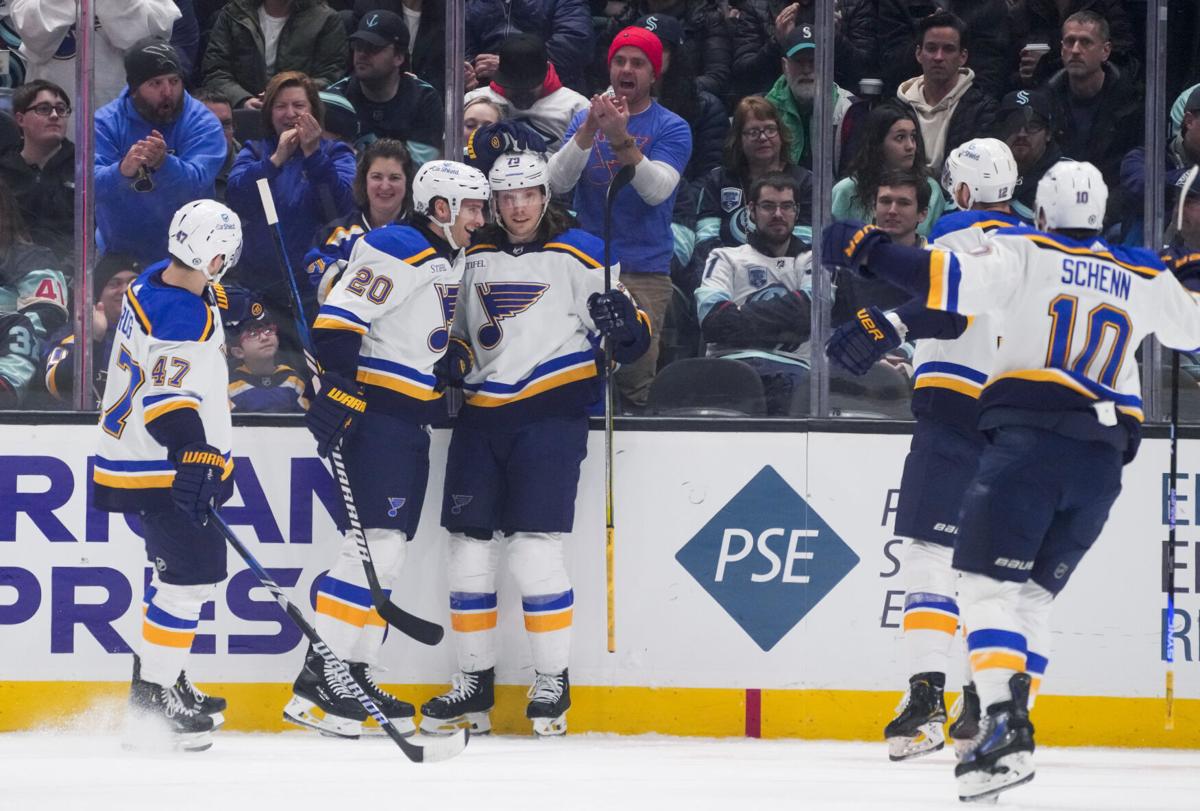In a vibrant full-color, square photograph captured indoors at a lively hockey match, five players from the same team are stationed on the ice amidst an intense game. Dressed in distinctive blue and white uniforms accented by a yellow stripe, and all wearing matching white helmets, these ice hockey players hold their sticks at the ready. The jerseys feature a design with blue shoulders, gold outlines, and white torsos, complete with coordinating white, yellow, and blue socks. Notably, player number 10, with the name SCHENN, faces away from the camera on the right, while numbers 47 and 80 appear on the left. The scene is set against a backdrop of a white barrier adorned with various writings, beyond which an enthusiastic audience claps and cheers. Positioned behind the clear plexiglass barrier, the fans, packed shoulder to shoulder, add to the dynamic atmosphere of the game.